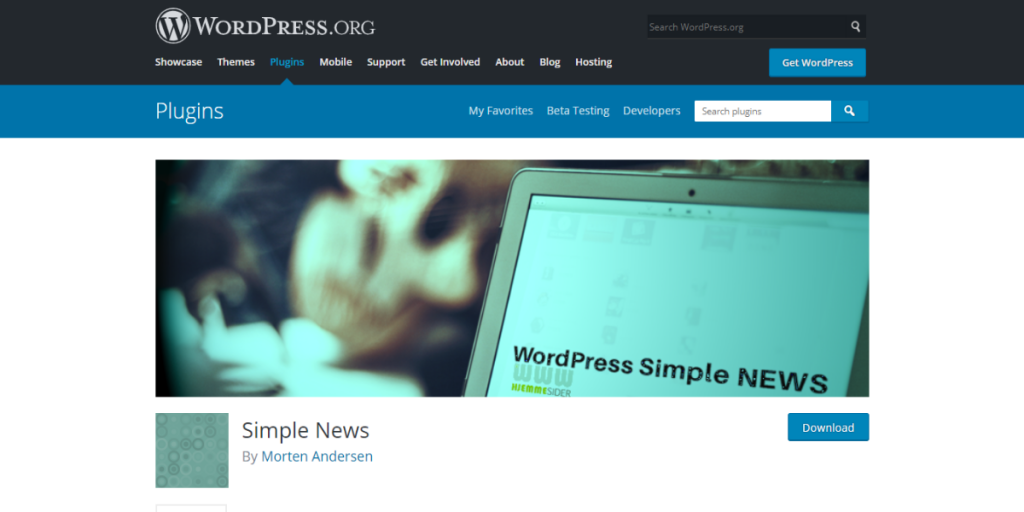The image depicts a webpage from WordPress.org, specifically the plugin section. At the top of the screen, the WordPress.org logo is visible on the upper left corner. A navigation menu features options such as Showcase, Themes, Plugins (highlighted in blue), Mobile Support, Get Involved, About, Blog, and Hosting, indicating clickable areas for various WordPress services and information.

On the upper right-hand side, there is a search icon and a text box labeled "Search WordPress.org". Adjacent to this, there's a "Get WordPress" button. Below this section, another search box, this time with the label "Search Plugins", is visible in white. To its left, links labeled "Developers," "Beta Testing," and "My Favorites" are displayed, suggesting areas that users can explore or click on.

Further down, there's a prominent image of a laptop screen showcasing "WordPress Simple News". Just below this, on the left-hand side, the caption reads "Simple News by Morton Anderson", while the right-hand side features a blue "Download" button. The midsection of the page displays a blurry, indistinct image, suggesting a focus on the Simple News plugin by Morton Anderson. 

Overall, the webpage provides a comprehensive layout of options, search functionalities, and highlighted features aimed at enhancing the user experience in navigating WordPress plugins.